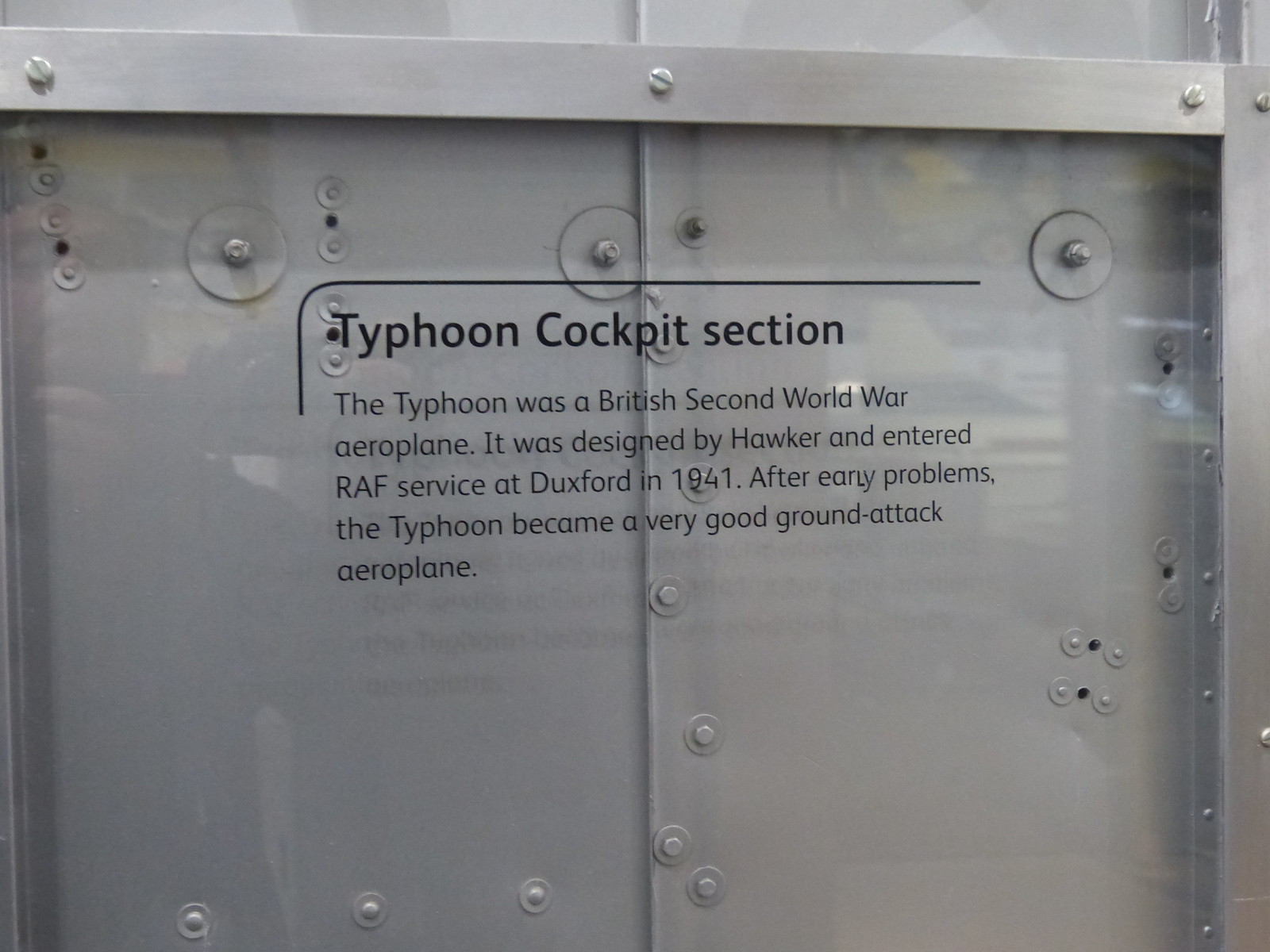The image shows a grey cockpit section of a Typhoon aircraft behind a glass panel, with numerous screws securing the metal panels. In the center of the image, large black text reads "Typhoon Cockpit Section," followed by a detailed paragraph in smaller black font. The text explains that the Typhoon was a British Second World War aeroplane designed by Hawker, entering RAF service at Duxford in 1941. Despite early issues, it eventually became an effective ground-attack aircraft. The reflective glass adds to the secure and preserved appearance of the display.